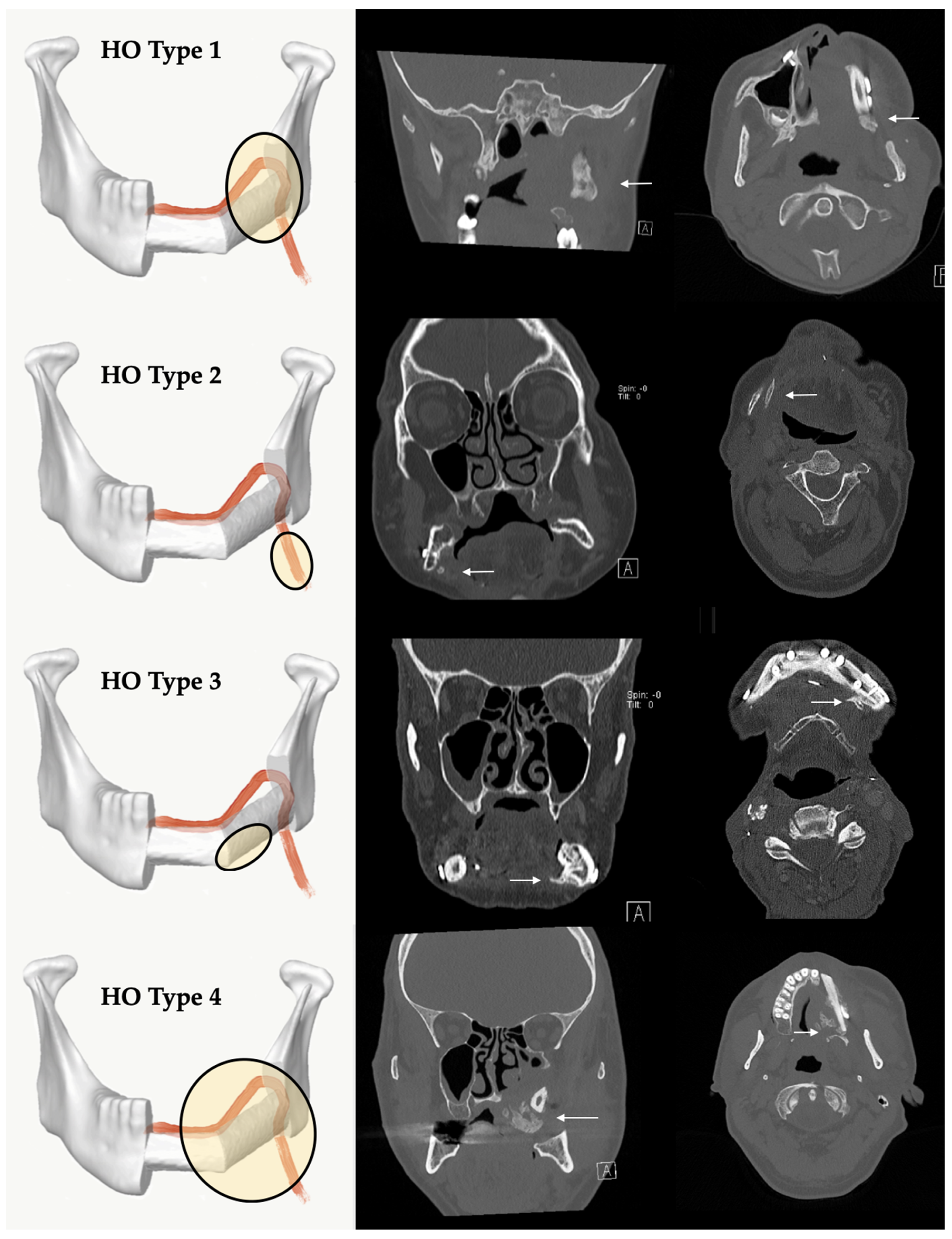The image is an educational material likely intended for medical students and professionals. It has a portrait orientation and is divided vertically into two sections. 

On the left-hand side, there is a white background featuring four detailed illustrations of jawbones, each labeled with "HO type" designations: HO type 1, HO type 2, HO type 3, and HO type 4. Each illustration highlights a specific area of the jaw with red markings, possibly indicating a nerve or tendon, and some sections are encircled in black rings with transparent yellow backgrounds for emphasis. The sequence appears to show different conditions or stages of an ailment affecting the jaw.

On the right-hand side, the background is black, displaying rows of what appear to be x-ray images or radiological drawings of the head and jaw. There are two columns of these grey-scale images, complete with various markings, abbreviations, and arrows, which are likely used for diagnostic purposes. The content suggests regions of medical interest that may require professional interpretation to understand fully.